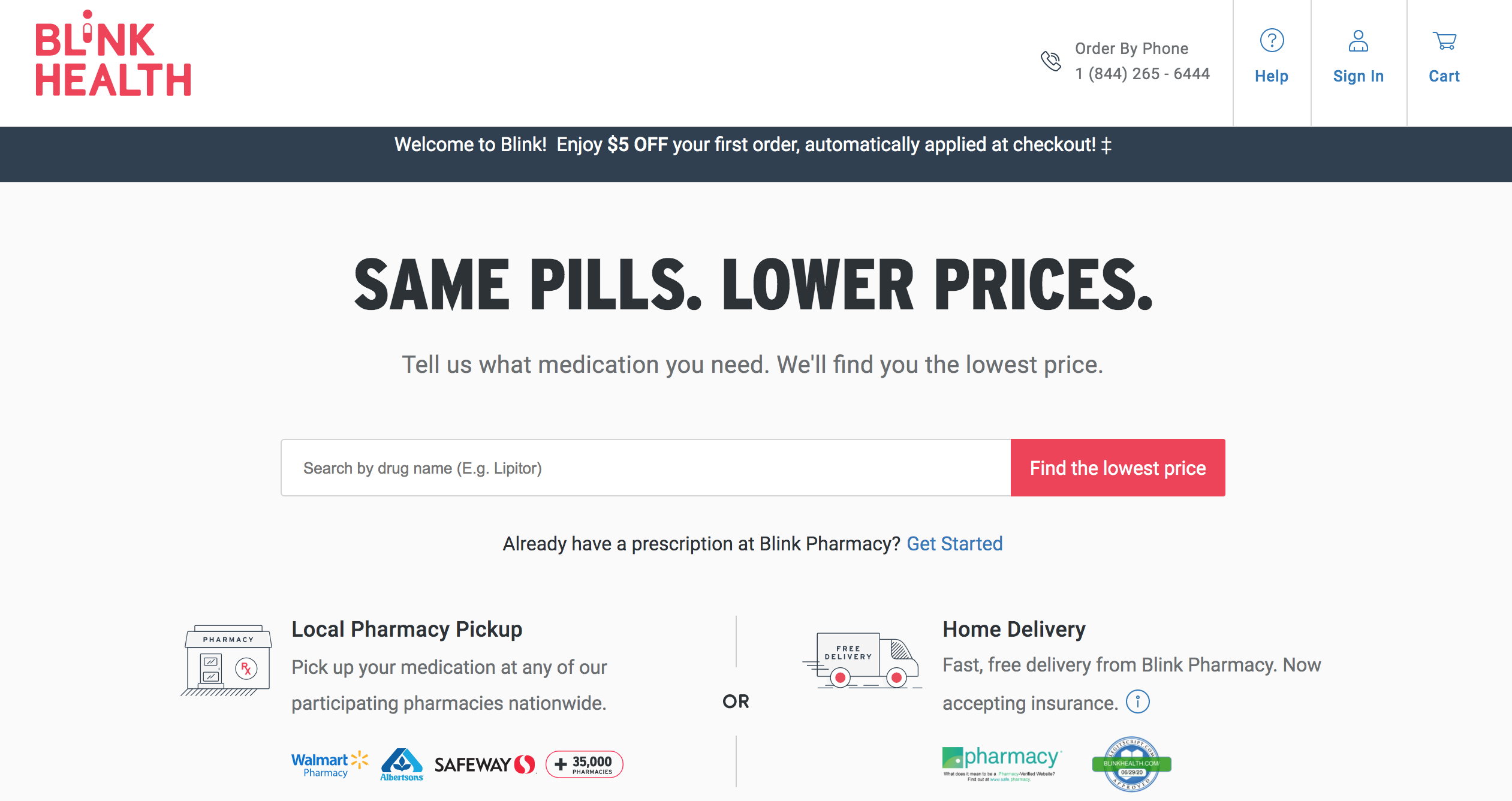In the image, a screenshot of the Blink Health website is depicted. At the top, there is a white border serving as a header. On the left of this border, the Blink Health logo is displayed. The logo features the text "Blink Health" with the "i" stylized to resemble a pill, split into two colors: the top half white and the bottom half pink.

On the far right of this top border, there is an "Order by Phone" section, featuring a phone icon and the number 1-844-265-6444 beneath. Next to this, a "Help" button with a blue, circled question mark icon is labeled "Help." Adjacent to it, an icon depicting a user profile (a simple head and shoulders outline) is labeled "Sign In." Further right, there is a shopping cart icon with the label "Cart."

Below the white top border, a thin, dark blue-gray line runs horizontally across the page. Centered within this line, in small white text, a welcome message reads: "Welcome to Blink. Enjoy $5 off your first order automatically applied at checkout."

The main content area of the page has a light gray background. At the top, a large heading in dark bluish-gray font states: "Same Pills, Lower Prices." Beneath this, in smaller, skinnier letters, a subheading reads: "Tell us what medication you need, we'll find you the lowest price." A search box is positioned below, pre-filled with example text: "Search by drug name (e.g., Lipitor)." To the right of the search box, a red button says "Find the Lowest Price" in white text.

Under the search box, a small black text prompts users with "Already have a prescription at Blink Pharmacy?" followed by a blue link stating, "Get Started." 

Below these prompts, there are two options for delivery methods. The first option is "Local Pharmacy Pickup," accompanied by a cartoon outline drawing of a pharmacy. Underneath this title, in small black letters, it says: "Pick up your medication at any of our participating pharmacies nationwide." Logos of participating pharmacies such as Walmart Pharmacy, Safeway, and others are displayed, including one with a blue triangle and a leaf design.

To the right of the "Local Pharmacy Pickup" section, the word "or" leads to the second option: "Home Delivery." This section features an outline drawing of a truck with "Free Delivery" written on it. Beneath "Home Delivery," small text reads: "Fast, free delivery from Blink Pharmacy, now accepting insurance." There is a small circle icon with what appears to be an exclamation point inside it.

Further down, two more icons are visible. One depicts a green square labeled "Pharmacy" in blue text, with some additional small text that is illegible. The other icon is a blue circle with a white border and a green rectangular box with white text running through the middle, though the text is not clear.

The detailed layout and organized sections aim to provide a user-friendly experience for visitors looking to order medications through the Blink Health platform.